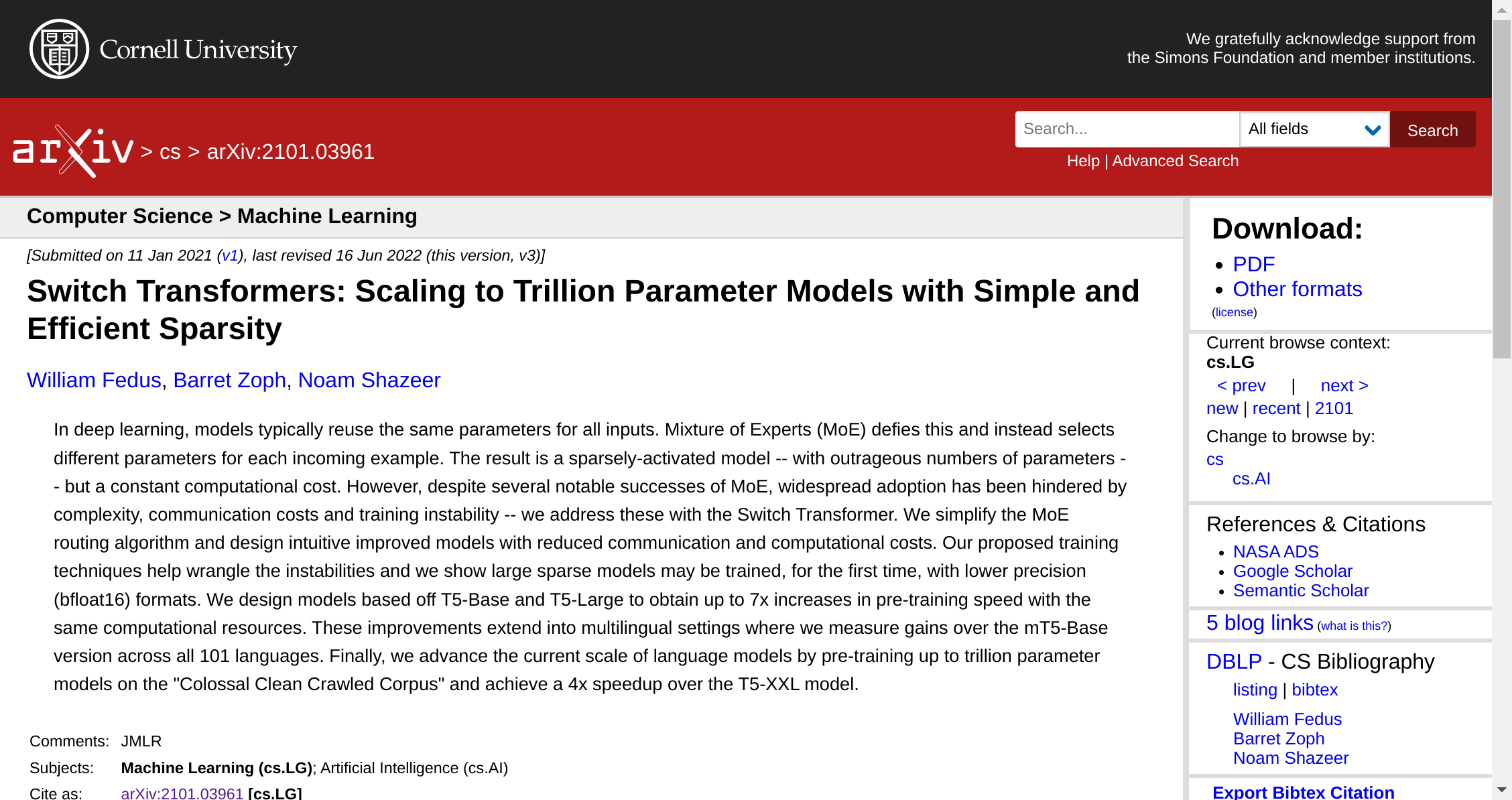The image features a sophisticated layout with several important elements. At the top, there is a sleek black border containing the words "Cornell University," along with a note expressing gratitude for support from the Simon Foundation and member institutions. Directly below this, a striking red box displays the text "arXiv:2101.03961."

Beneath the red box, there's a search interface that includes a drop-down menu labeled "All fields," next to a prominent "Search" button. Moving further down, text indicates the category: "Computer Science > Machine Learning," followed by submission information noting that the paper was initially submitted on January 11, 2021, and last revised on June 16, 2022. This current document version is noted as "v3."

The title of the paper, "Switch Transformers: Scaling to Trillion Parameter Models with Simple and Efficient Sparsity," is clearly marked. The authors are listed as William Thaddeus, Barrett Zopf, and Noam Shazir. A brief abstract suggests that the study discusses deep learning models that typically reuse the same parameters for input, and introduces the concept of a mixture of experts that instead selects different parameters.